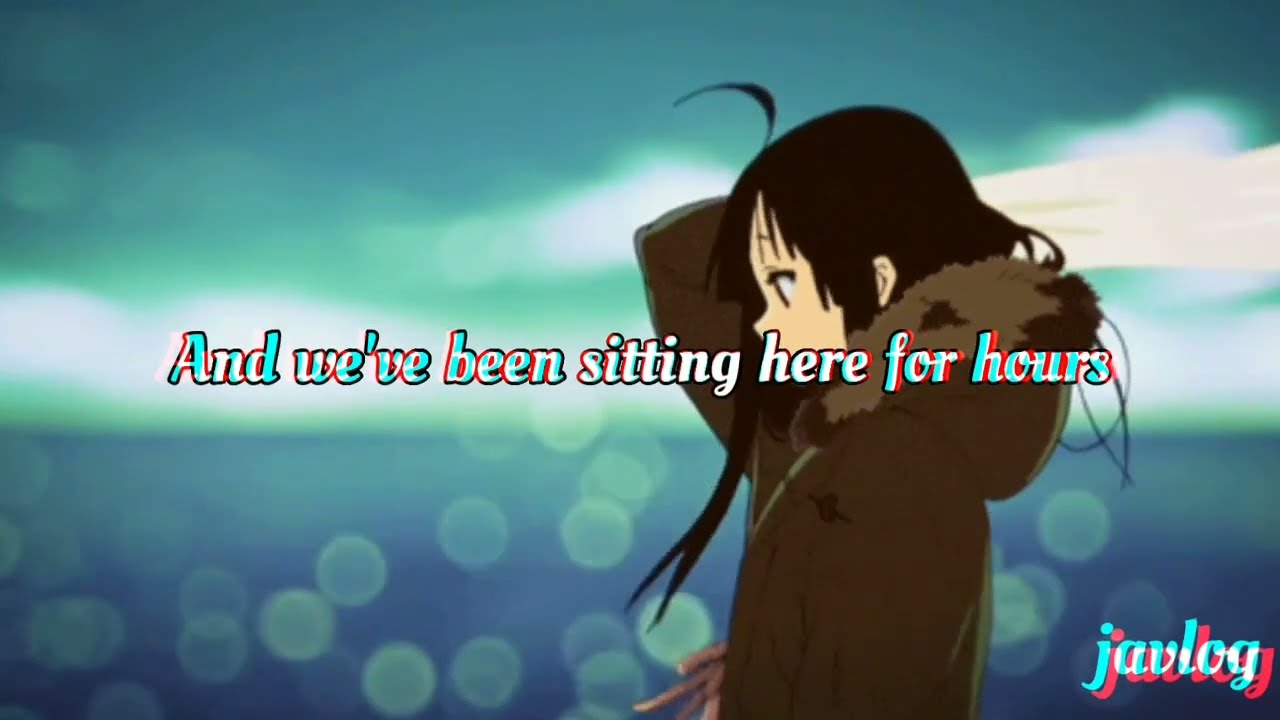The digital artwork is a wide rectangular piece featuring an anime-style girl situated slightly to the right of center. She is depicted in a side profile facing left, with long, straight black hair and her head tilted downwards, eyes gazing towards the ground. She wears a heavy brown winter coat, complete with a furry hood that rests behind her head. The girl has white skin and her posture conveys a sense of contemplative melancholy.

The background is a blurry depiction of a deep bluish-turquoise body of water, plastered with neon green, transparent polka dots that mimic the appearance of bubbles. Above this, the sky is a rich turquoise, dotted with clouds that have neon green outlines and white centers. The horizon line is positioned roughly one-third of the way up the image, suggesting a serene, albeit abstract landscape.

Overlaying this scene in white bubble letters with chromatic aberration effect, the text reads, "and we've been sitting here for hours." Another piece of white text with the same chromatic aberration effect, "J-A-V-L-O-G," is located in the bottom right-hand corner. The overall ambiance of the artwork combines elements of digital surrealism with a touch of introspective stillness from the central character.